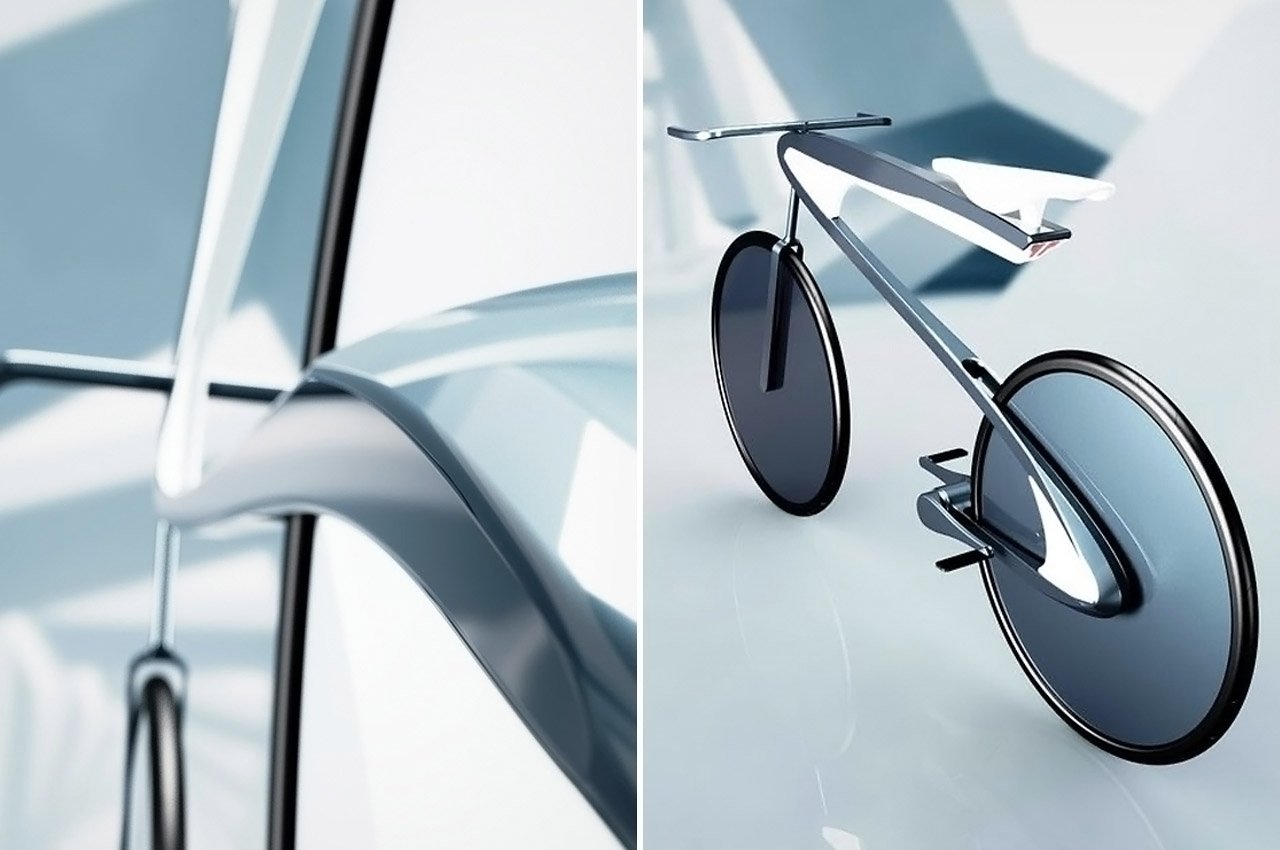The image showcases a futuristic bicycle set against a gray background. The right half of the image features the full side view of the bike, characterized by its sleek, straight frame, a white Z-shaped seat, transparent wheels with a light green tint where the spokes should be, and minimalist pedals resembling crank sticks. The bicycle appears to be computer-generated, with a metallic silver and green color scheme enhancing its avant-garde appeal. The left half of the image zooms in on a specific part of the bicycle, likely the handlebar area, which is challenging to identify precisely due to its abstract, close-up presentation. This section also displays a transparent appearance with a black frame running through it, continuing the futuristic and polished design language seen throughout the bicycle.